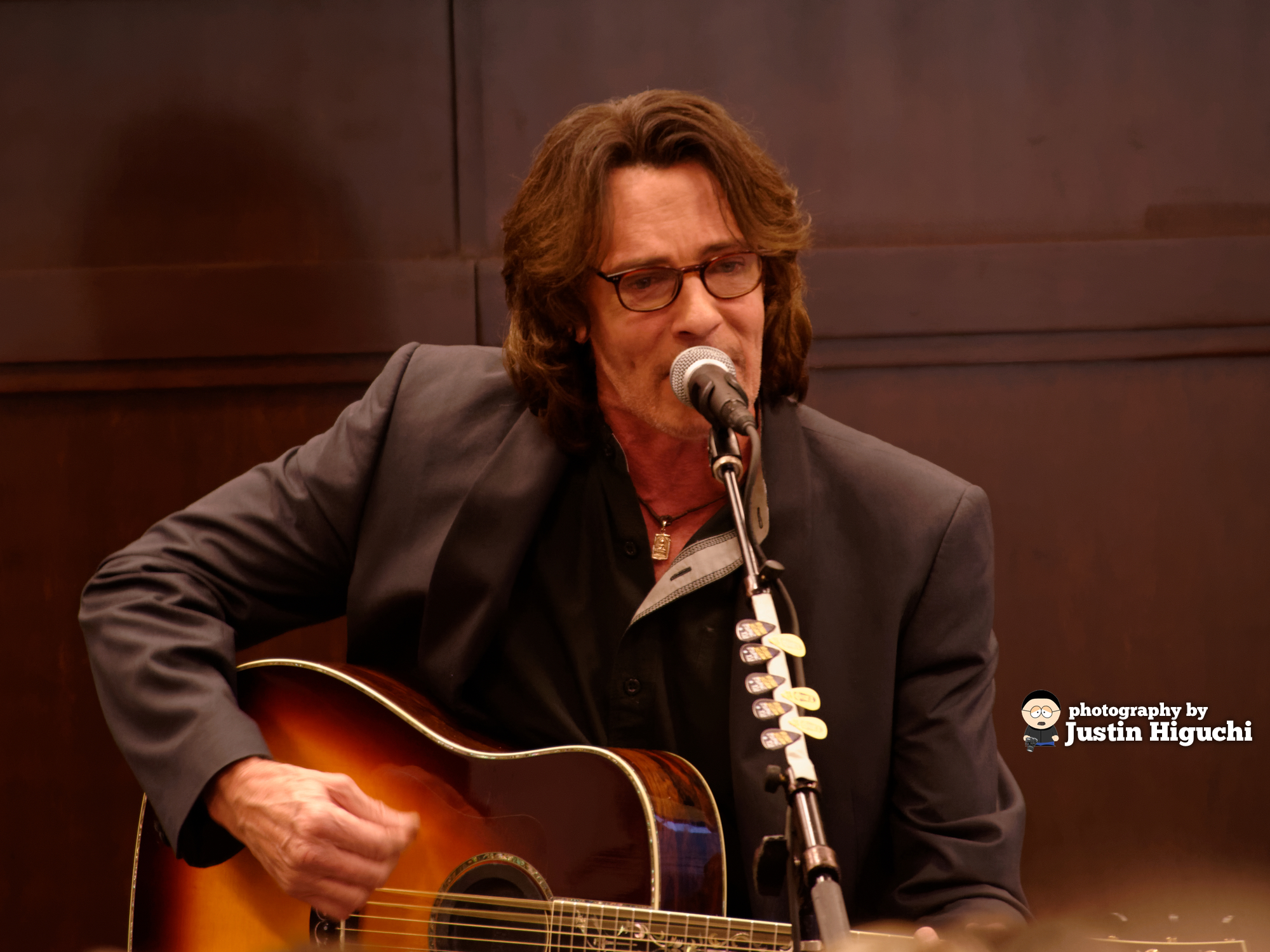In the photograph, a man is captured sitting at the center, viewed from his stomach upwards. He is attired in a black business coat over a black button-up shirt with the top two buttons left undone, revealing a black necklace with a rectangular gold pendant. His face, framed by shoulder-length brown hair, is adorned with black-rimmed glasses. He holds a light brown and dark brown acoustic guitar; his left hand is engaged with a guitar pick, and his right hand grasps the guitar's neck. Positioned before him, a black microphone stand with a silver-tipped microphone aimed at his face is visible, its black wire trailing down the stand. The backdrop is a brown wooden wall. In the bottom right corner, text reads "photography by Justin Higuchi." For additional information, www.FEMA.gov is noted. The setting appears to depict an indoor musical performance. The image showcases a palette of brown, gray, tan, silver, and gold tones.